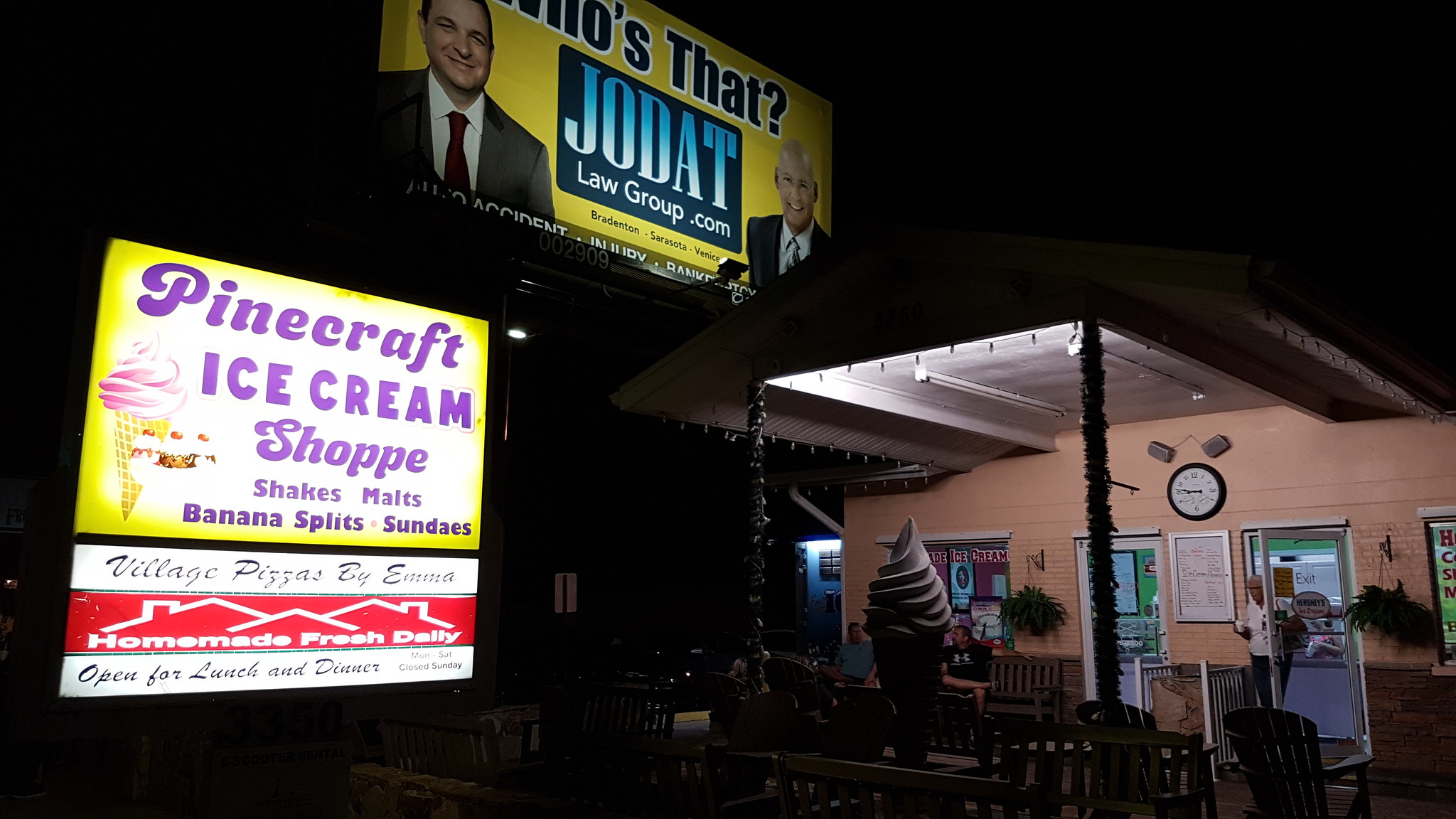The photograph, taken at night, captures the front of the Pinecraft Ice Cream Shop, a small, warmly lit establishment with a little canopy over the entryway. A customer is seen exiting the shop with something in hand. Adjacent to the main door is another entrance framed by a small wall with a plaque, flanked by windows. The shop's inviting exterior is complemented by a colorful image of an ice cream cone, indicating its specialty. To the left, a large, illuminated sign advertises an array of treats including shakes, malts, banana splits, and sundaes, with a narrower sign below promoting Village Pizzas. Dominating the scene above these signs, a massive billboard displays an advertisement for "Jodablawgroup.com" featuring two figures and prominently showcasing yellow text. The bright lights from the billboard illuminate the area, highlighting a few patrons lined up outside, eager to purchase ice cream.